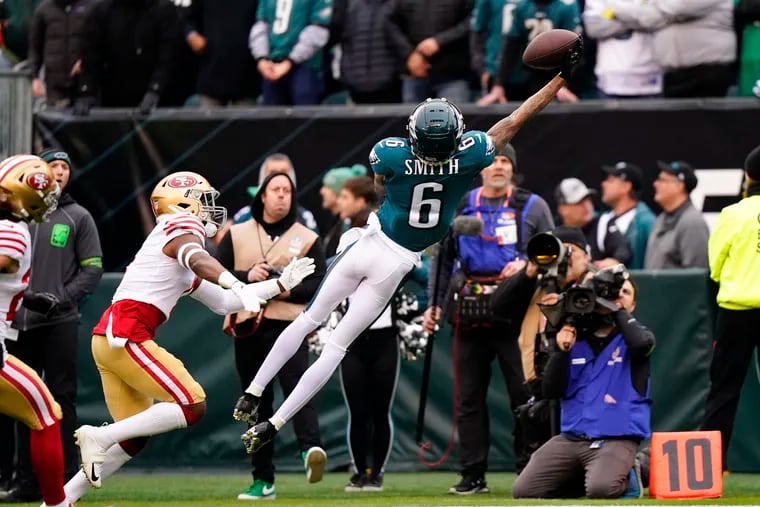In this photograph from the 2022 NFC Championship game between the Philadelphia Eagles and the San Francisco 49ers at Lincoln Financial Field, we see a dramatic moment where Eagles wide receiver DeVonta Smith, in action mid-air, reaches out with his right hand to catch the football. Smith is wearing white pants, black cleats, a green jersey with white lettering reading "Smith 6," and a green helmet adorned with white wings on the sides. Chasing him are two San Francisco 49ers players dressed in white jerseys with red undershirts, gold pants featuring red and white stripes, gold helmets with red "SF" emblems, and white cleats, one of whom is also wearing red socks.

In the background, Eagles fans are discernible, with a mix of fans, support staff, and photographers clad in a variety of colored jackets, including black and gray, with some wearing neon yellow jackets. Near the right edge of the image, a cameraman dressed in blue is kneeling to record the scene, with another cameraman positioned slightly higher behind him. An orange yard marker bag displaying the number 10 is also visible. Among the bystanders, one individual with an open mouth looks on, capturing the intensity and excitement of this pivotal play, which contributed to the Eagles' victory in the game.